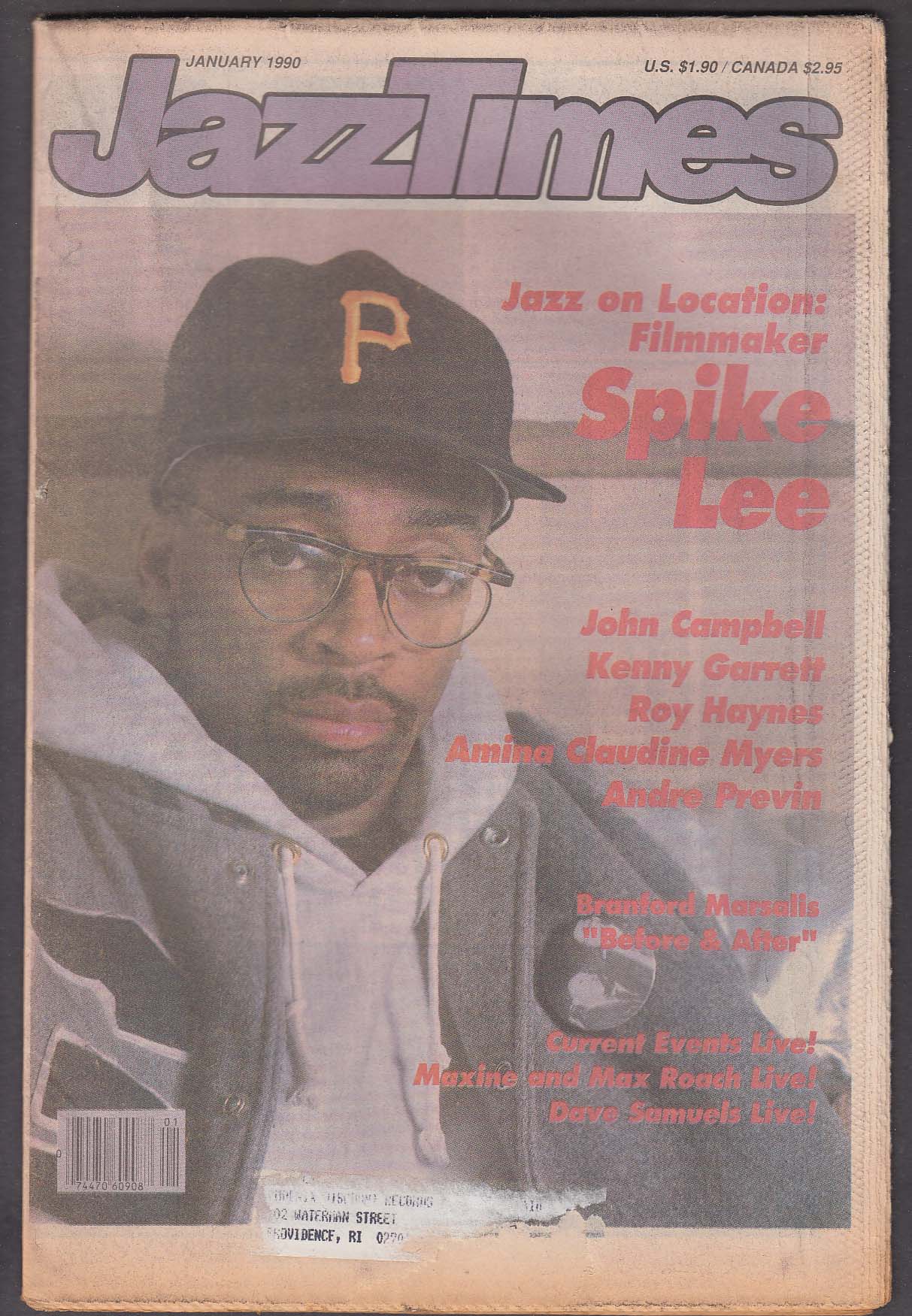This image features the front cover of a vintage publication titled "Jazz Times" from January 1990, priced at $1.90 in the U.S. and $2.95 in Canada. The cover, which has muted and somewhat faded colors, prominently displays its title in large purple, bubbly font. Below the title, the cover showcases a photograph of African-American filmmaker Spike Lee, distinguishable by his glasses, cap with a yellow 'P', French beard, gray hoodie, and green jacket.

On the right side of Spike Lee's image, a series of headlines in red font lists notable personalities and features including Jazz on Location with Filmmaker Spike Lee, John Campbell, Kenny Garrett, Roy Haynes, Amina Claudine Myers, Andre Previn, Branford Marsalis, as well as articles like Before and After, Current Events Live, Maxine and Max Roach Live, and Dave Samuels Live.

The bottom left corner of the magazine cover contains a barcode, number 7447060908. Centrally at the bottom, there's a partially ripped-off white and black address label, with legible fragments reading 'Waterman Street', 'Providence, R.I., 0270'. The overall layout is well-organized, despite the off-center elements, maintaining a balanced and appealing aesthetic suitable for a magazine cover.